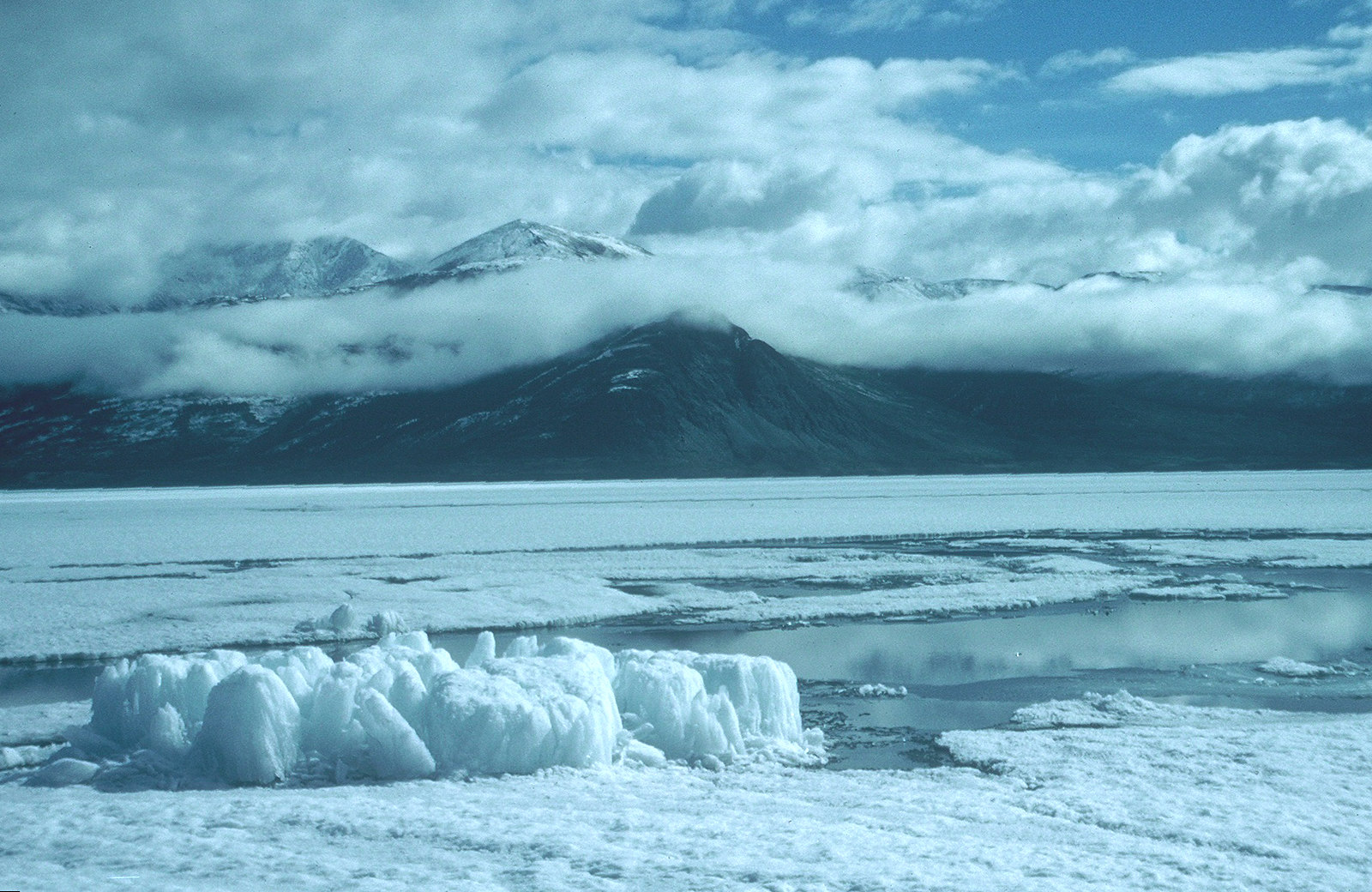A stunning photograph of the Arctic landscape features a snow-capped mountain in the distant background, towering majestically. In the foreground, a starkly contrasting dark mountain looms, devoid of snow, accentuating the desolate beauty of the scene. The expanse between the mountains is covered in vast sheets of ice and snow, with small icebergs dotting the frigid terrain. A narrow strip of water winds its way between the ice sheets, adding a sense of movement to the frozen tableau. Overhead, the sky is a light shade of blue, partially obscured by numerous clouds that hang low, mingling with the peaks. The entire vista is bathed in a serene mixture of white snow, the deep black of the mountain, and the soft hues of the sky, creating a dramatic and mesmerizing Arctic panorama.